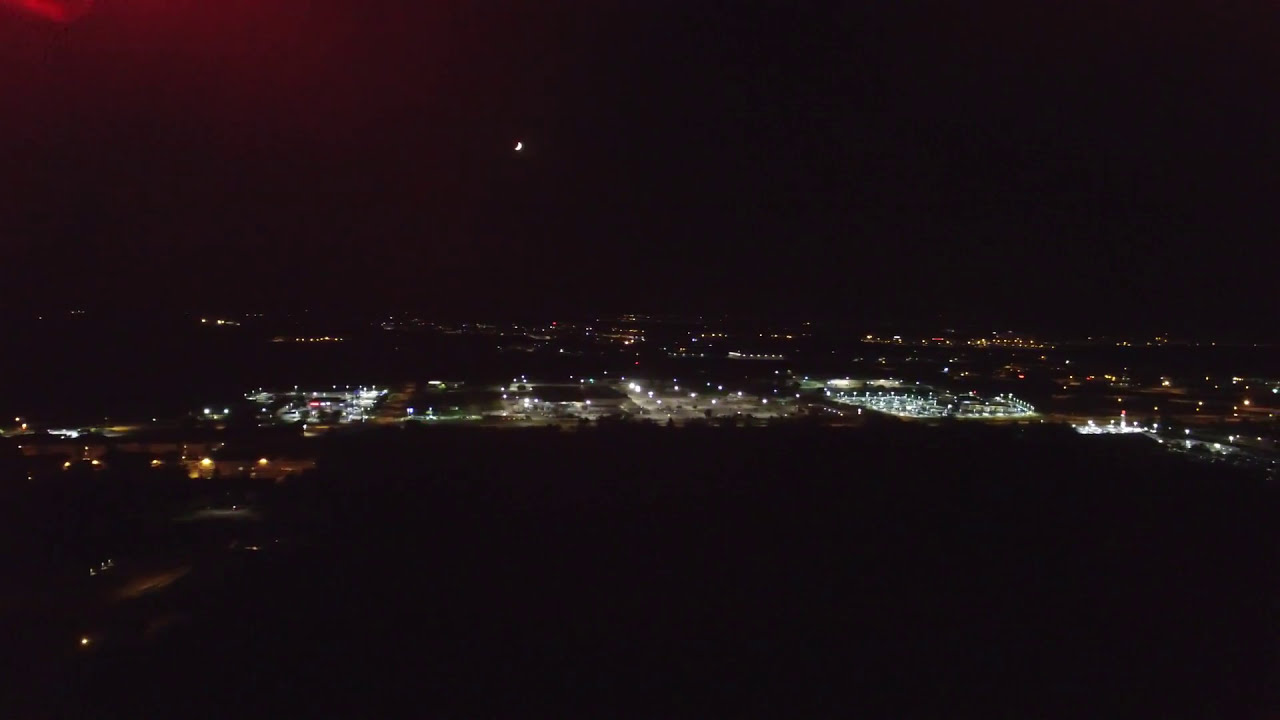This is a horizontal rectangular aerial photograph taken at night. The vast majority of the image is shrouded in darkness, dominated by shades of black. In the upper portion of the image, there is a small, bright white dot that appears to be a crescent moon, situated slightly to the left of the center. Below this, the horizon of the Earth is visible, revealing a field of city lights stretching across the middle section of the photograph. The lights are predominantly the sodium vapor orange color, interspersed with patches of brighter white lights, especially in clusters. Toward the right side of the image, an area is illuminated intensely, suggesting the presence of a stadium, with a faint touch of green hinting at possibly grass or turf. The majority of the lighted area in the image appears to be city lights, likely residential or commercial areas, forming a sea of tiny dots against the black backdrop. Towards the bottom and edges of the photograph, there is a larger expanse of darkness, which could signify areas of vegetation or water, though details remain obscured due to the nighttime setting. The only discernible colors in the image are black, white, yellow, and faint green.